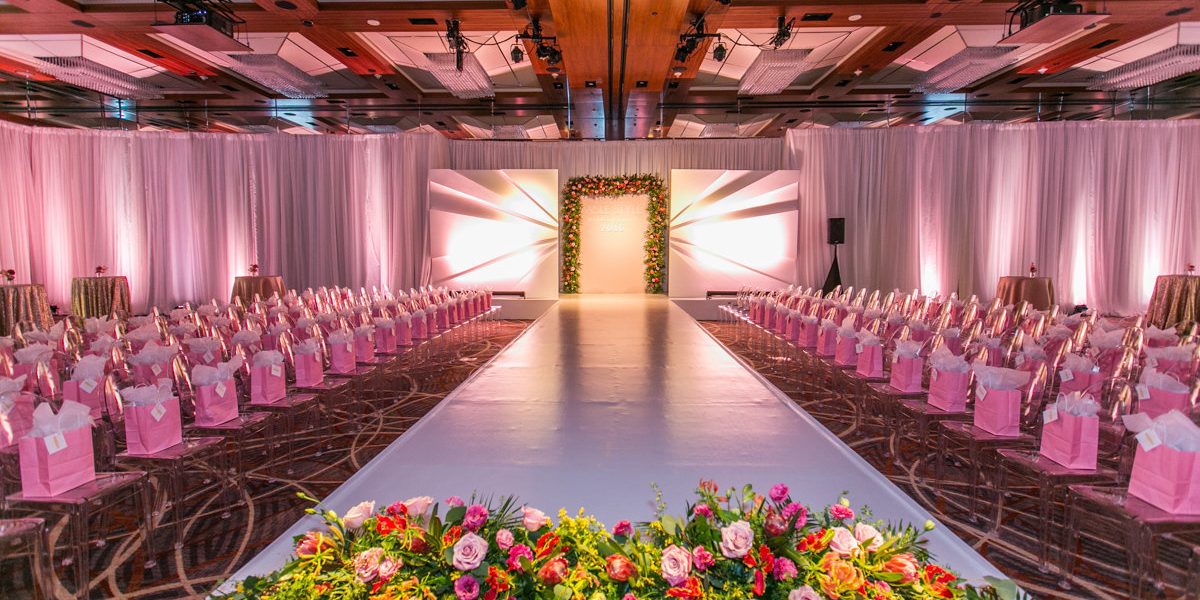The photograph captures a meticulously arranged, long room set for a high-society fashion show. The centerpiece of the room is a sleek, light gray runway extending forward from the vantage point, flanked by three rows of dark-colored chairs on either side. Each chair is adorned with a pink gift bag containing white tissue paper and a small card. At the photographer's end of the runway, bright and colorful flower arrangements in shades of orange, pink, yellow, and green create a vibrant foreground.

The backdrop of the room is defined by luxurious, pinkish-purple drapes that hang from the ceiling to the floor, illuminated by drop lights shining upward. Further enhancing the ambiance, intricate floral swags and canvases with radiant white orbs and pink and purple hues frame a doorway at the far end of the runway, suggesting an entry point for models. Overhead, industrial white fluorescent fixtures and black stage lighting provide ample illumination, casting a soft glow across the entire setting.

The walkway itself is bordered by an ornate carpet with light-colored swirl patterns, visible only in glimpses due to the numerous arranged chairs. Behind these seating arrangements are circular tables draped in metallic pinkish-purple fabric, each crowned with flower centerpieces, adding to the room's overall aesthetic elegance. This pre-event scene, awaiting the arrival of guests, exudes a sense of anticipation and sophistication.